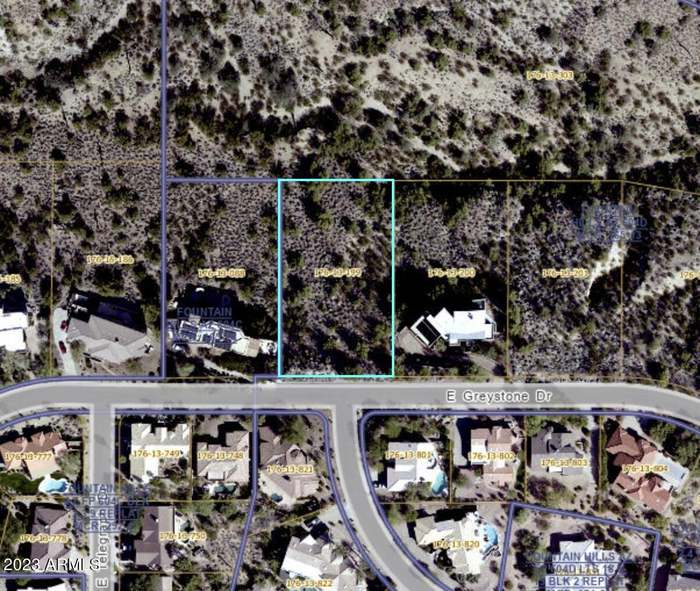The image is an aerial view of a residential neighborhood map, accentuated by both natural and digital elements. At the top, the map displays a densely forested, hilly area with sparse open ground visible through the tree cover. Below this natural zone, the map transitions into a developed area, marked by colored lines—purple, blue, and yellow—likely denoting property or zoning boundaries. Across the bottom half of the image runs East Greystone Drive, a prominent gray street that stretches horizontally. Two roads branch off this main street: one curves from the middle and the other diverges from the front left, labeled East Telegraph. Interspersed around these roadways are numerous houses, each marked with what appears to be latitude and longitude coordinates. Additionally, rectangular regions indicate specific property lots. A faint purple watermark and a label reading "2023 ARMI Space S" are also visible, indicating the image's digital overlay.